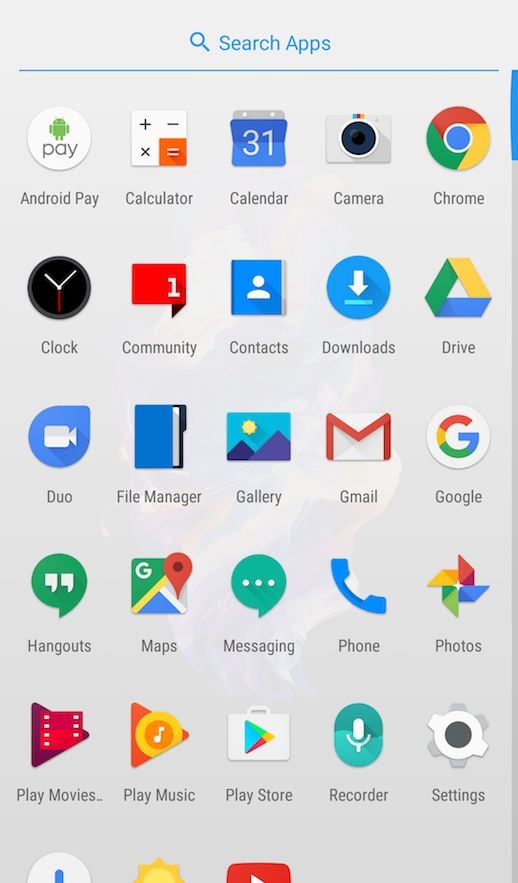A detailed image caption of an Android phone's app drawer displaying pre-installed applications:

The screenshot showcases the app drawer of an Android phone, dominated by a neutral light grey background. At the top of the screen, there's a prominent search bar labeled "Search apps," accompanied by a magnifying glass icon, facilitating quick app searches. The app drawer reveals a comprehensive list of pre-installed applications, arranged in a grid format. The visible apps include Android Pay, Calculator, Camera, Chrome, Clock, Community, Contacts, Downloads, Drive, Duo, File Manager, Gallery, Gmail, Google, Hangouts, Maps, Messaging, Phone, Photos, Play Movies, Play Music, Play Store, Recorder, and Settings. Towards the bottom of the list, a few apps are partially visible, suggesting that Weather and YouTube are among them, along with one unidentified app. This eclectic mix consists of both circular and irregularly shaped icons, indicating no strict uniformity in icon design—only a requirement to fit within a specified space. Notably, the presence of older applications like Hangouts hints at the phone's age, inferring it might be an older Android model. The minimal user customization suggests the device is either newly set up or owned by someone with minimal app usage needs.